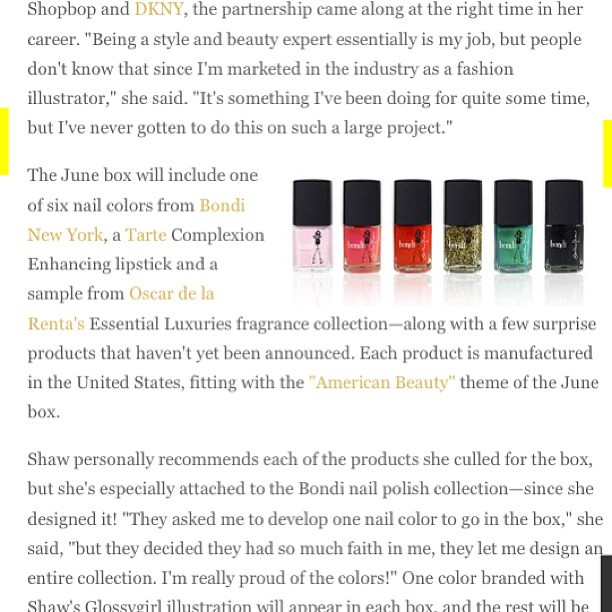This image is a detailed screenshot of an article from a beauty website, prominently featuring text about a collaboration between Shopbop and DKNY. The text explains that the partnership came at an opportune moment in Shaw's career, a style and beauty expert who is typically known in the industry as a fashion illustrator. She expresses excitement about working on a larger scale project, having curated and designed products for the June beauty box. The box will include one of six nail colors from Bondi, New York, a Tarte complexion-enhancing lipstick, and a sample from Oscar de la Renta's Essential Luxuries fragrance collection, among other surprise products. Shaw specially recommends the Bondi nail polish collection, which she designed herself. The visible nail polish bottles feature black lids and come in various colors such as pink, hot pink, red, gold glitter, aqua green, and black. The aesthetic of the image suggests that it is a clipping from an online beauty article, emphasizing text over visuals. The products mentioned are American-made, aligning with the June box's American beauty theme.